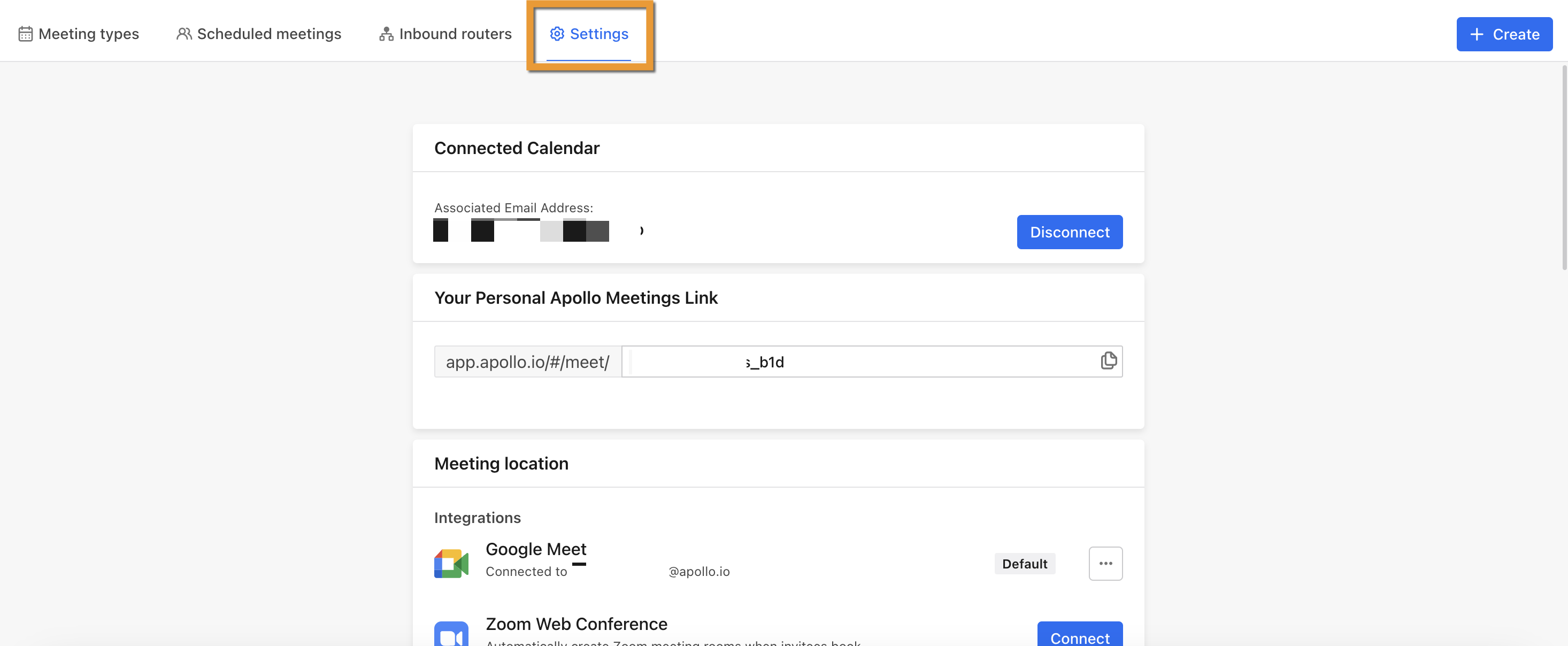The screenshot captures the settings page of a Google-related account, displayed in a rectangular format. The layout is wider than it is tall. At the very top, a thin white navigation bar extends horizontally from the left to the right. This banner presents three main selectable options in black text: "Meeting Types," "Scheduled Meetings," and "Inbound Routers." Additionally, there are two interactable buttons on this banner. On the far right side is a blue rectangular button labeled "Create" in white text.

Moving toward the center of the top banner, to the left of the "Create" button, a setting item is highlighted with blue text reading "Settings" accompanied by a small cog icon to its left. An orange border surrounds this setting, drawing attention to it.

The main body of the page is light gray. Centrally positioned are three white rectangular sections. The topmost rectangle is titled "Connected Calendar" at its top. Inside this section, there is text indicating an "Associated Email Address." The actual email address has been obscured using various colored squares.